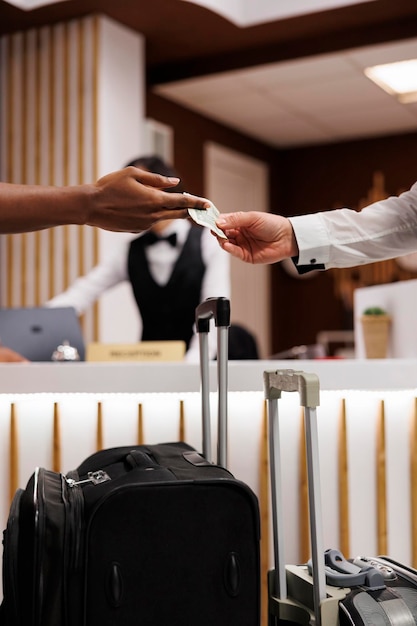In this highly detailed vertical image, a cash exchange is taking place, suggesting a tip being given in a hotel or possibly an airport lounge setting. In the foreground, the top halves of two suitcases are visible—one black and one silver—standing next to each other with their handles prominent. Above the luggage, two hands are making the exchange: the arm on the right, wearing a white sleeve, extends cash to a darker-skinned hand on the left, which grasps the money between its pointer and middle finger. The background features a person in formal attire—a white shirt with long sleeves under a black vest and a bow tie—working at a Mac computer on a desk. A nameplate also sits on the desk in front of them. The environment, with black walls and white ceilings accented by a white wall with gold stripes, hints at an indoor, formal setting such as a hotel lobby.